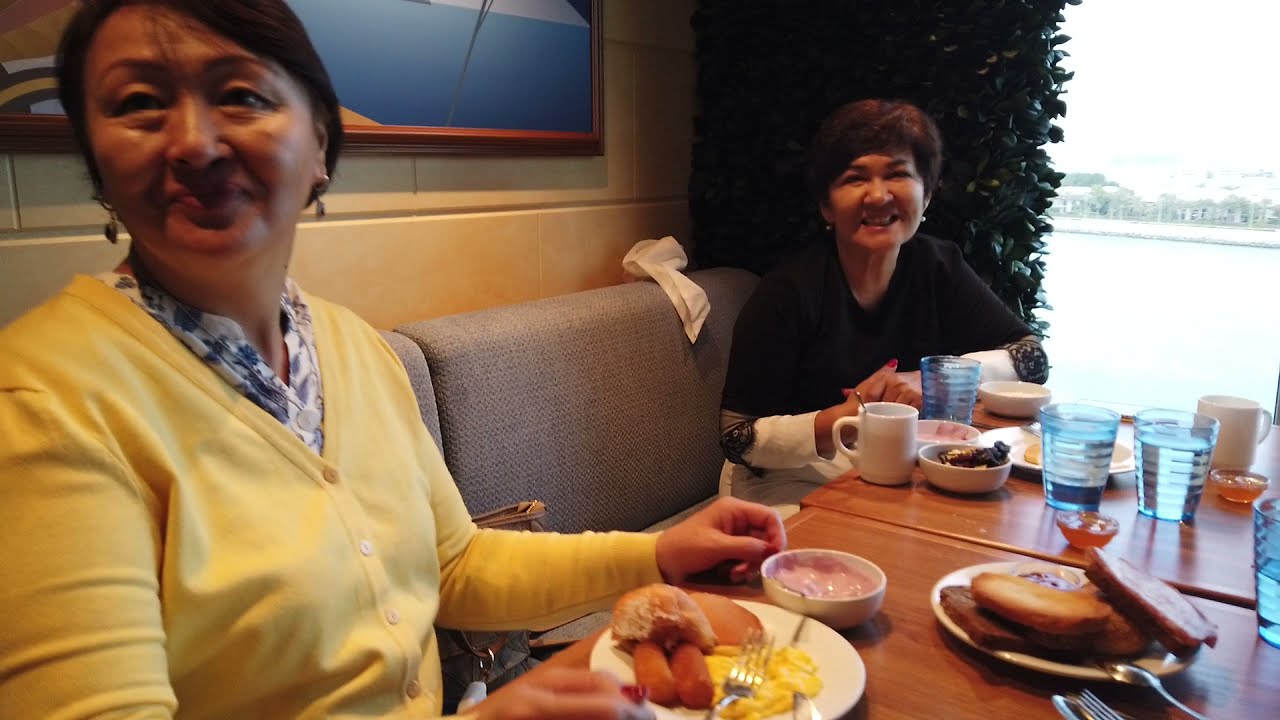In this detailed image, two women of possible Asian descent, perhaps Japanese, are seated in a restaurant booth with gray seats. They are likely mother and daughter. To the left, the woman is wearing a yellow button-down sweater over a blue and white blouse, paired with silver earrings. She has dark hair and appears to be in her 40s, looking toward the camera but not directly at it. On the right, the other woman, also likely in her 40s, wears a black and white sweater with white pants and silver earrings. She is smiling and looking more directly at the camera, her hands folded on the table. 

The booth they sit in is by a window with a blurry daytime view outside, and behind them, the wall is yellow, possibly tiled, with a green plant near the lady in black and a multicolored picture in a reddish-brown or cherry wood frame near the lady in yellow. There is also a brown purse beside her.

In front of them on the brown table are several breakfast items. The centerpiece is a large plate of toast, accompanied by four blue glasses of water and two white coffee cups. The woman in yellow has a bowl of what appears to be strawberry yogurt, a plate with eggs and a roll, and a big plate of toast in the middle of the table. The other woman has a bowl with what seems to be blackberries or possibly blueberries. Both women also have white plates featuring breakfast foods like eggs, sausage, and possibly pancakes. A white towel or napkin is visible behind the woman in black.